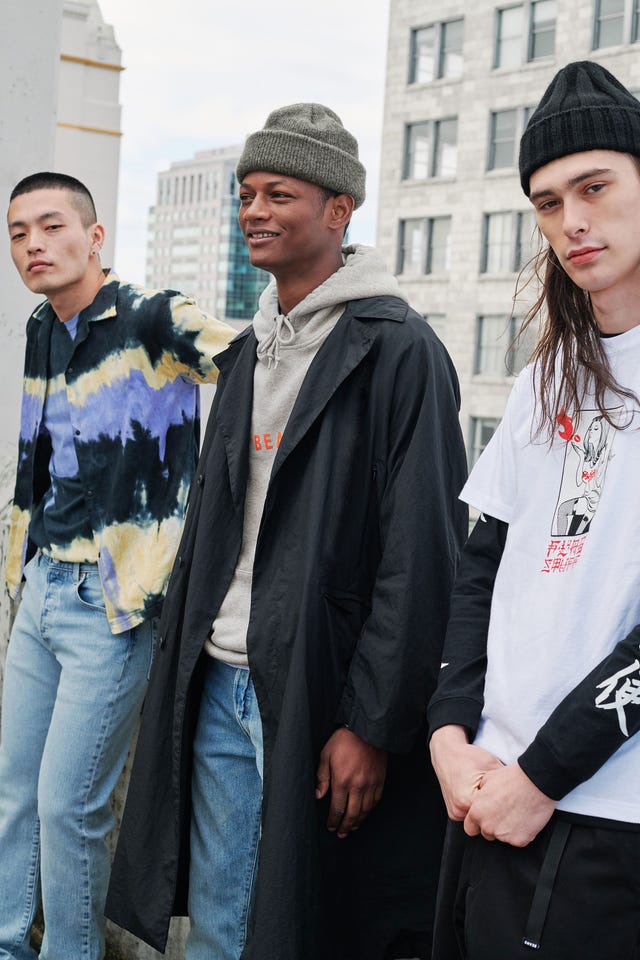This detailed digital photograph captures three young men—each distinguished by their ethnicities and unique attire—posing on a rooftop against a backdrop of high-rise buildings. The man on the right, who appears younger and is likely engaged in parkour, is Caucasian. The central figure, clad in a black cape or robe, is black, while the man on the left, who looks Asian, sports a distinctive shirt adorned with blue, cream, and light-colored hues, along with white blue jeans. The scenery boasts an urban skyline with several high-rise buildings featuring white and gold trims and teal-colored windows, adding contrast to the primarily black, gray, white, and blue tones of the photograph. Text in a different language is also visible within the image, enriching its cultural context.